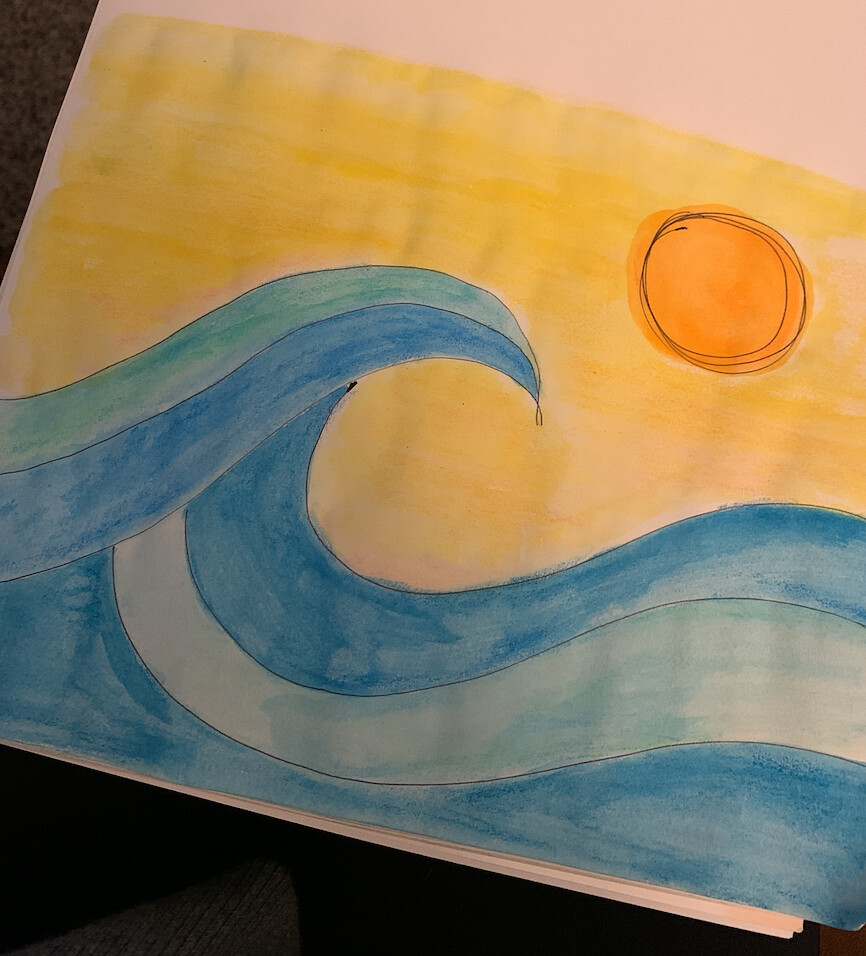This charming illustration, rendered with a blend of pencil or pen and subsequently filled in with watercolor, exudes a whimsical, childlike quality. The focal point of the artwork is a stylized wave, depicted in a medley of dark blue, light blue, and bluish-green hues, giving it a dynamic and vibrant appearance. Above the wave stretches a vivid yellow sky that radiates warmth and energy. Dominating the sky is an orange Sun, uniquely characterized by scribbled circular motions that create a textured, playful effect. This piece captures the exuberance and innocence of a child's imagination brought to life on paper.